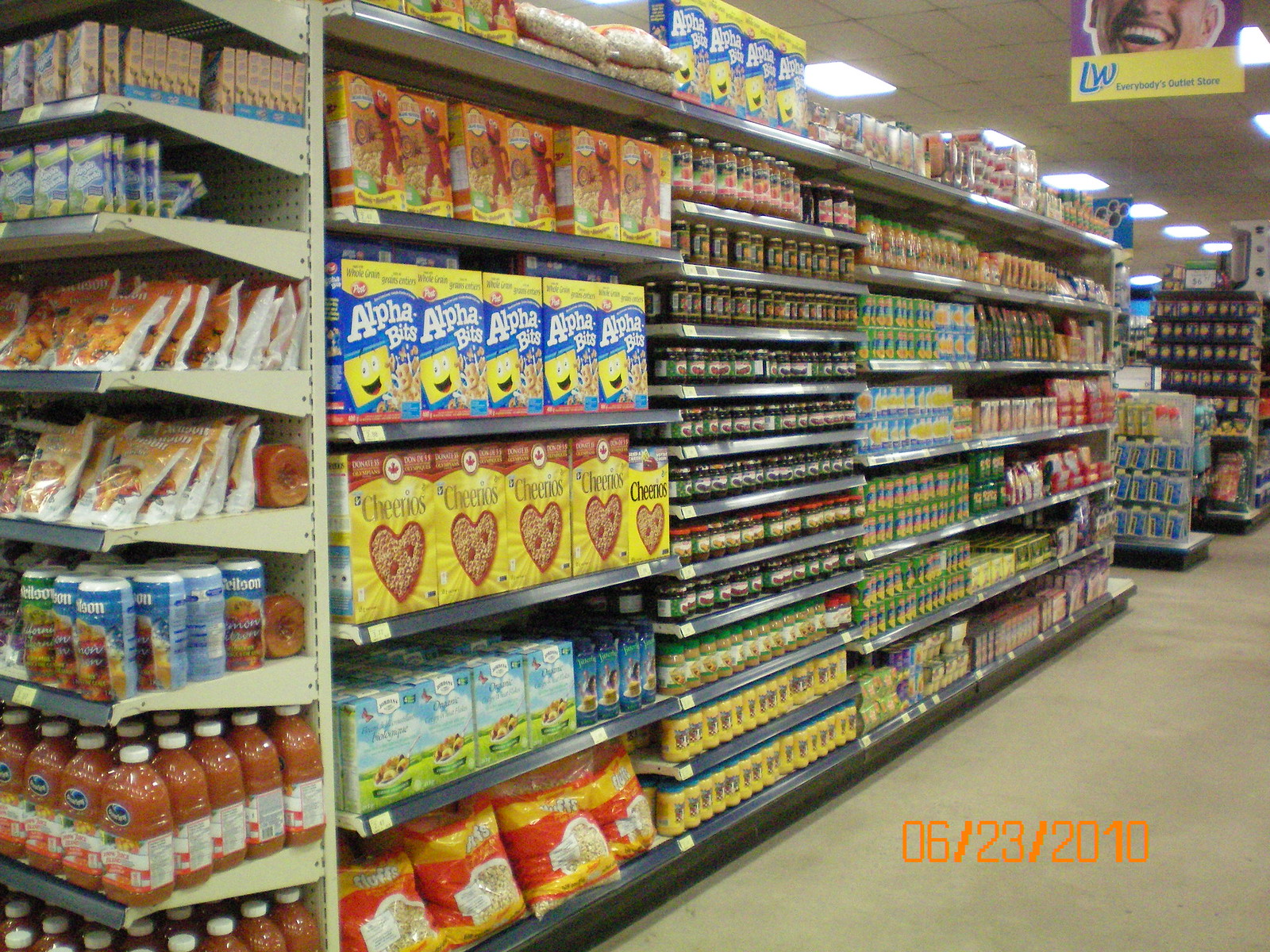This image depicts a supermarket aisle extending from the left foreground to the right-hand upper background, showcasing a meticulously organized and well-stocked section. The supermarket floor is a polished, smooth grey concrete. In the bottom right corner of the photograph, the date "06/23/2010" is prominently displayed in orange text. 

The aisle features an array of shelves filled with various breakfast and other packaged food items. The bottom shelf near the end of the aisle is packed with large bags of oats, suitable for breakfast. As our eyes move upwards, the next shelves are populated with an array of cereals, including well-known brands like Cheerios and Alphabits, along with another cereal endorsed by Elmo. Above the cereals, some shelves hold smaller packages resembling jelly crystals.

Further along the aisle, the stocked products shift to spreads, such as jams and potentially applesauce, and canned fruits. Jars of different food items are visible, illustrating a diverse selection of breakfast-related products. Additionally, there are possible boxed drinks aligning the rest of the shelving, adding to the variety of items available. Overhead, the aisle is illuminated by rectangular lights fitted within a suspended ceiling grid, emphasizing the well-lit, welcoming environment of the supermarket.